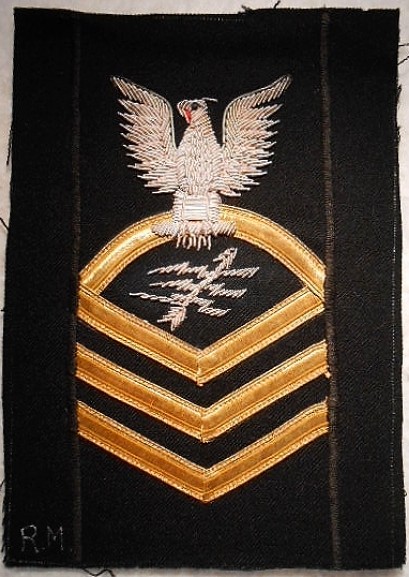This colored photograph features an up-close image of a frayed military emblem patch with a black background and white trim. Prominently in the center, there is a stitched white eagle with its wings spread wide, seemingly holding something in its beak. Directly beneath the eagle is a white arrow intersected by three lightning bolts. Below the arrow is a curved gold piece, followed by three gold V-shaped stripes that peak downwards. The initials "RM" are visible in white stitching in the lower left-hand corner of the patch. The patch appears to be placed against a white surface, adding contrast to its intricate details and slightly worn edges.